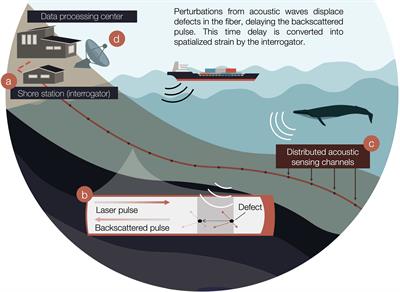This scientific cartoon illustrates the process of distributed acoustic sensing (DAS) using a fiber optic system submerged in an ocean environment. At the top, black lettering explains: "Perturbations from acoustic waves displace defects in the fiber, delaying the backscattered pulse. This time delay is converted into specialized strain by the interrogator." The scene features a simplistic tanker ship on the ocean surface emitting black sound waves, suggesting the source of perturbations. Below the sea level, a whale is depicted emitting white sound waves, further illustrating acoustic interactions.

In the lower portion of the image, a red and brown box labeled "C" reads "distributed acoustic sensing channels," highlighting how these channels capture the acoustic signals. To the left, another box labeled "B" displays "laser pulse, backscattered pulse, and defect," along with diagrams of the respective waves to visually represent the data collection process. In the top left corner, a small cartoon building with a satellite dish, marked "A and B," is labeled "data processing center" and "shore station interrogator," indicating where the collected data is processed and analyzed.

The image effectively combines multiple graphical elements to convey the complex process of how acoustic waves interact with fiber optic sensors to detect and measure underwater disturbances.